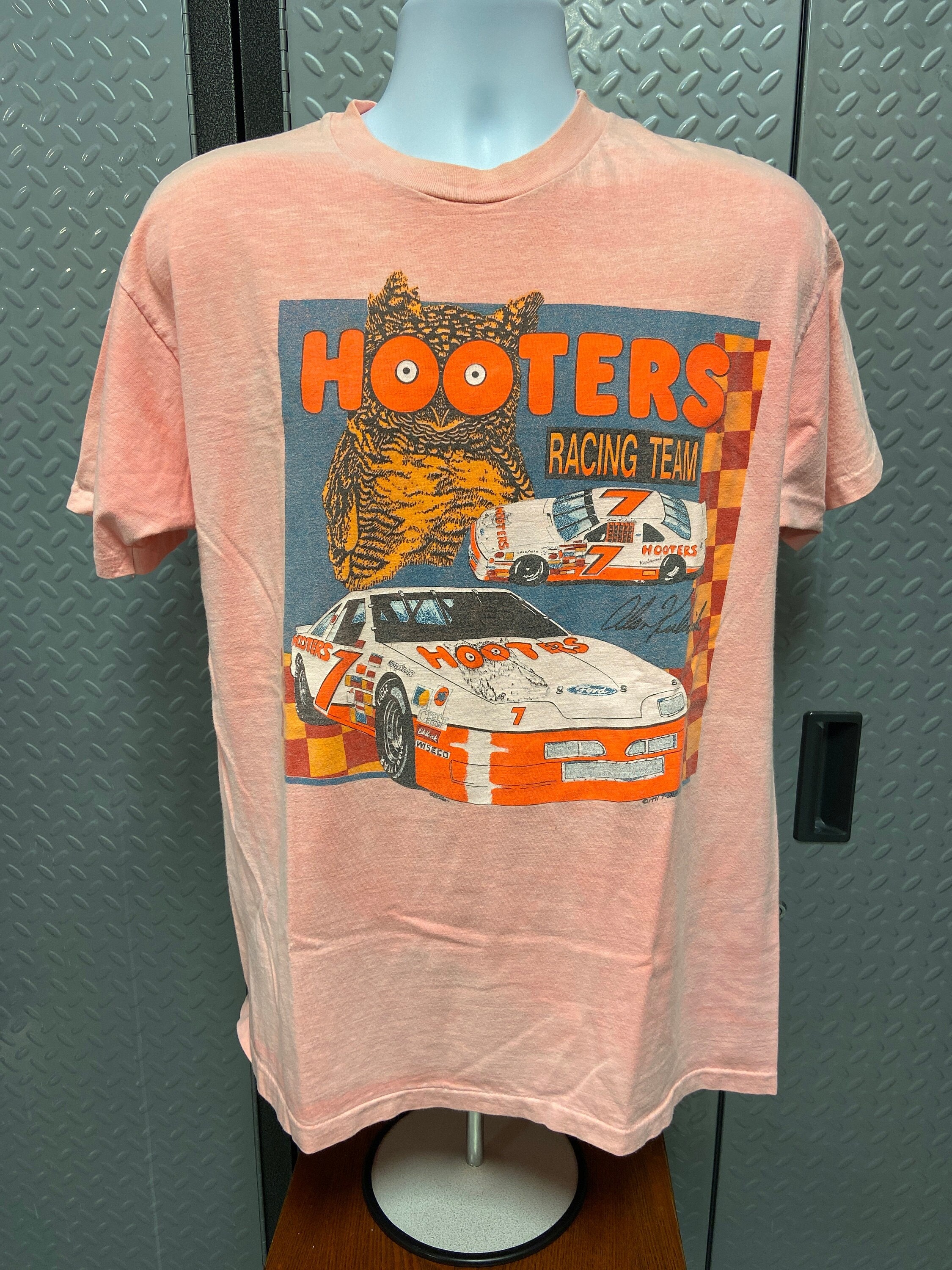This is an image of a grayish beige half-mannequin on a metal stand, sitting on a brown wooden table in front of gray metal lockers with black handles and an embossed crosshatch design. The mannequin wears a salmon pink t-shirt, faded to a peach hue, promoting the popular Hooters restaurant and its racing team. The shirt features a large Hooters logo in bright orange with the iconic owl whose eyes form the O's in "Hooters." Below the logo, it says "Racing Team" in an orange and white bar. The centerpiece is a blue square background displaying two images of the number seven Hooters race car – one front view and one side view – both white with orange detailing and the Hooters branding. Behind the blue square, there is a checkered flag design in burgundy and mustard gold, enhancing the racing theme of the t-shirt.